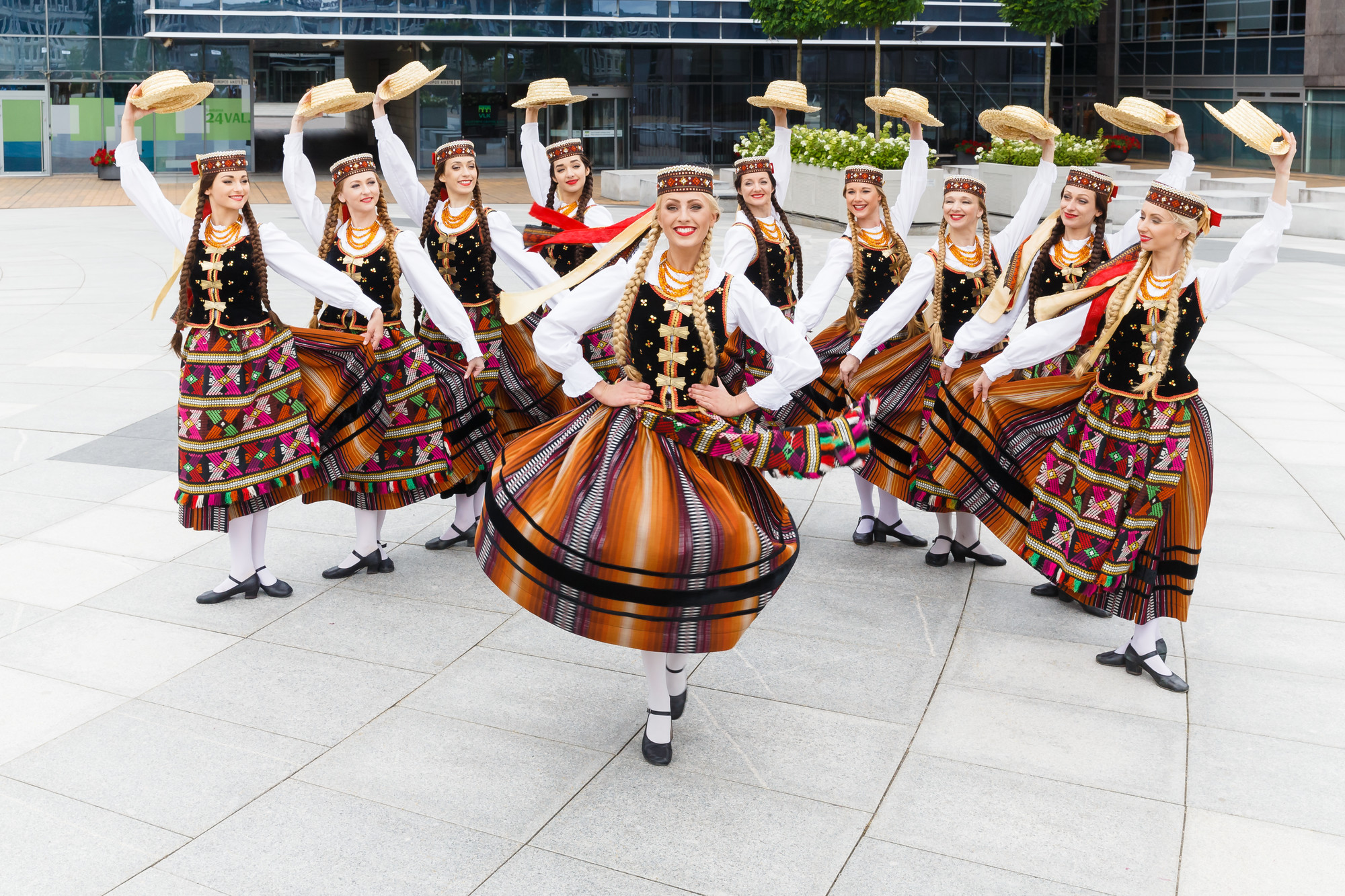The photograph features a group of 10 women dressed in traditional Eastern European or Hungarian attire, gathered in a modern city plaza in front of a corporate building with a sign reading "24VAL." The central woman is the focal point, smiling with her hands on her hips. She has long blonde hair styled in two front braids, adorned with a traditional straw hat. Her dress includes a black bodice with four bows, a white collared shirt, and a skirt with orange and burgundy stripes. The other nine women, positioned 4 on her left and 5 on her right, mirror her traditional outfit and hairstyle. Each of them raises a flat, brimmed straw hat above her head, suggesting they are preparing for a dance performance. The concrete plaza is dotted with planters filled with white flowers, adding a touch of nature to the urban setting. Their coordinated poses and festive attire indicate a sense of unity and anticipation for a cultural dance performance.